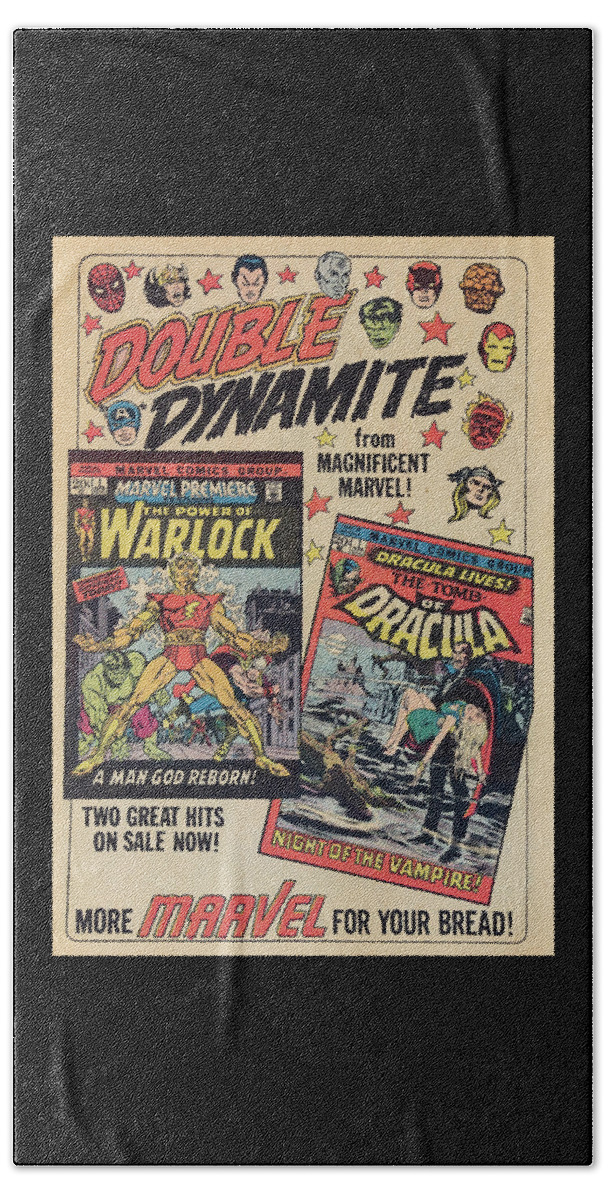This is a detailed promotional poster for vintage Marvel comic books. At the top, in bold comic book lettering, the words "Double Dynamite" are prominent, with "Double" in orange and "Dynamite" in black. Surrounding this headline are small, iconic headshots of various Marvel characters, including Spider-Man, Iron Man, Thor with his Viking helmet and long blonde hair, Daredevil, The Thing, The Incredible Hulk, and Captain America. Below the headline, it notes that this is from "Magnificent Marvel." The poster prominently features two comic book covers side by side— "The Power of Warlock" and "The Tomb of Dracula." The "Power of Warlock" cover is orange, while "The Tomb of Dracula" is black, both with bold yellow titles. At the bottom of the poster, it enticingly claims, "Two great hits on sale now," followed by the slogan, "More Marvel for your bread," suggesting these thrilling comic books are must-buys for enthusiasts. The entire design suggests it is an advertisement likely seen in the 1950s, possibly displayed in storefronts to attract comic book fans.